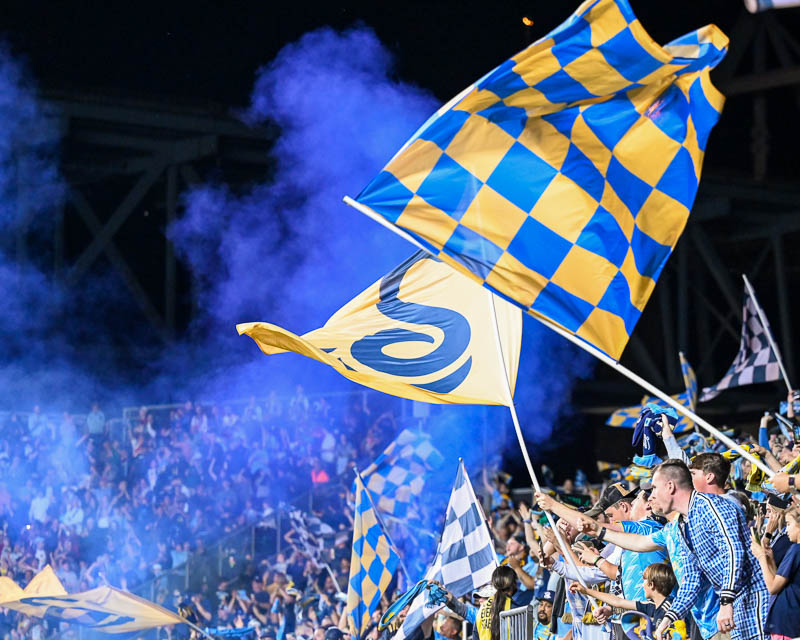The image captures a vibrant and energetic scene at a large sporting event, possibly a racing event or a European professional football match, given the prevalence of checkerboard flags and the celebratory atmosphere. The packed bleachers teem with a diverse crowd of men, women, and children, all engrossed in the event. Many fans wave flags of various designs: some with the traditional black and white checkered pattern typical of race car events, others in striking blue and yellow, and a notable yellow flag adorned with a black squiggly line resembling a snake. There's also a flag with a blue logo, likely representing the sports team. The stands are filled to capacity, with no empty seats in sight, and the air is thick with white smoke, possibly from race cars or celebratory flares. Enthusiastic fans can be seen clapping, cheering, and capturing the moment with their cell phones. A man in the bottom right wears a distinctive white and blue checkered sweatsuit, further adding to the dynamic and colorful ambiance of the event.